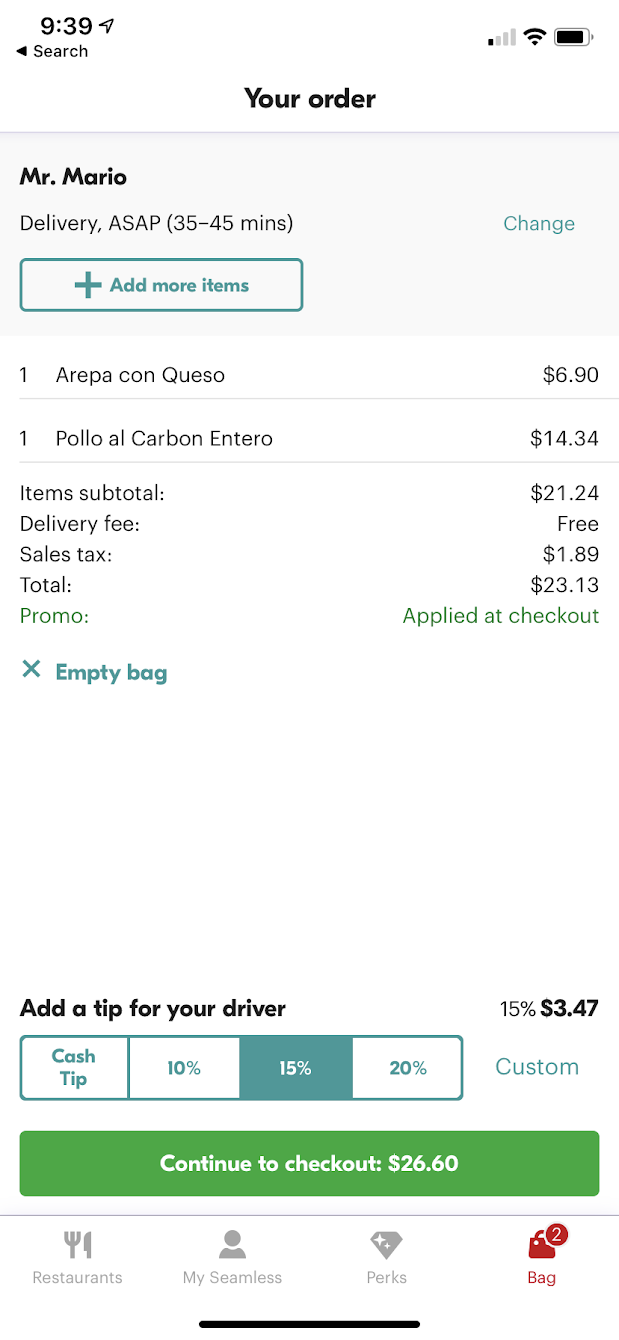Here is a detailed and cleaned-up caption for the image:

---

This image is a screenshot of a delivery order page displayed on a cell phone. At the top center, the page is titled "Your Order." Just beneath this title, in a light gray box, the name "Mr. Mario" is displayed in bold text. Below the name, it states "Delivery ASAP 35 to 45 minutes," with an option to "Change" this displayed in blue on the right side.

On the left side of the screen, there is a rectangular button labeled "Add More Items." Below this button, the ordered items are listed: "One Arepa con Queso $6.90" and "One Pollo al Carbón and Taro $14.34." The item's subtotal is shown as "$21.24," followed by "Delivery Fee: Free" and "Sales Tax: $1.89," bringing the total to "$23.13." A note indicates "Promo Applied at Checkout."

On the left, there is an "X" with the option to "Empty Bag." Further down, the page prompts the user to "Add a Tip for Your Driver," highlighting a 15% tip, equating to "$3.47," in bold. Tip options include "Cash Tip," "10%," "15%," "20%," with the 15% option highlighted, and an additional "Custom" option.

At the bottom of the page, a large green button labeled "Continue to Checkout $26.60" is prominently displayed. The bottom navigation bar features four icons labeled "Restaurants," "My Seamless," "Perks," and "Bag."

---